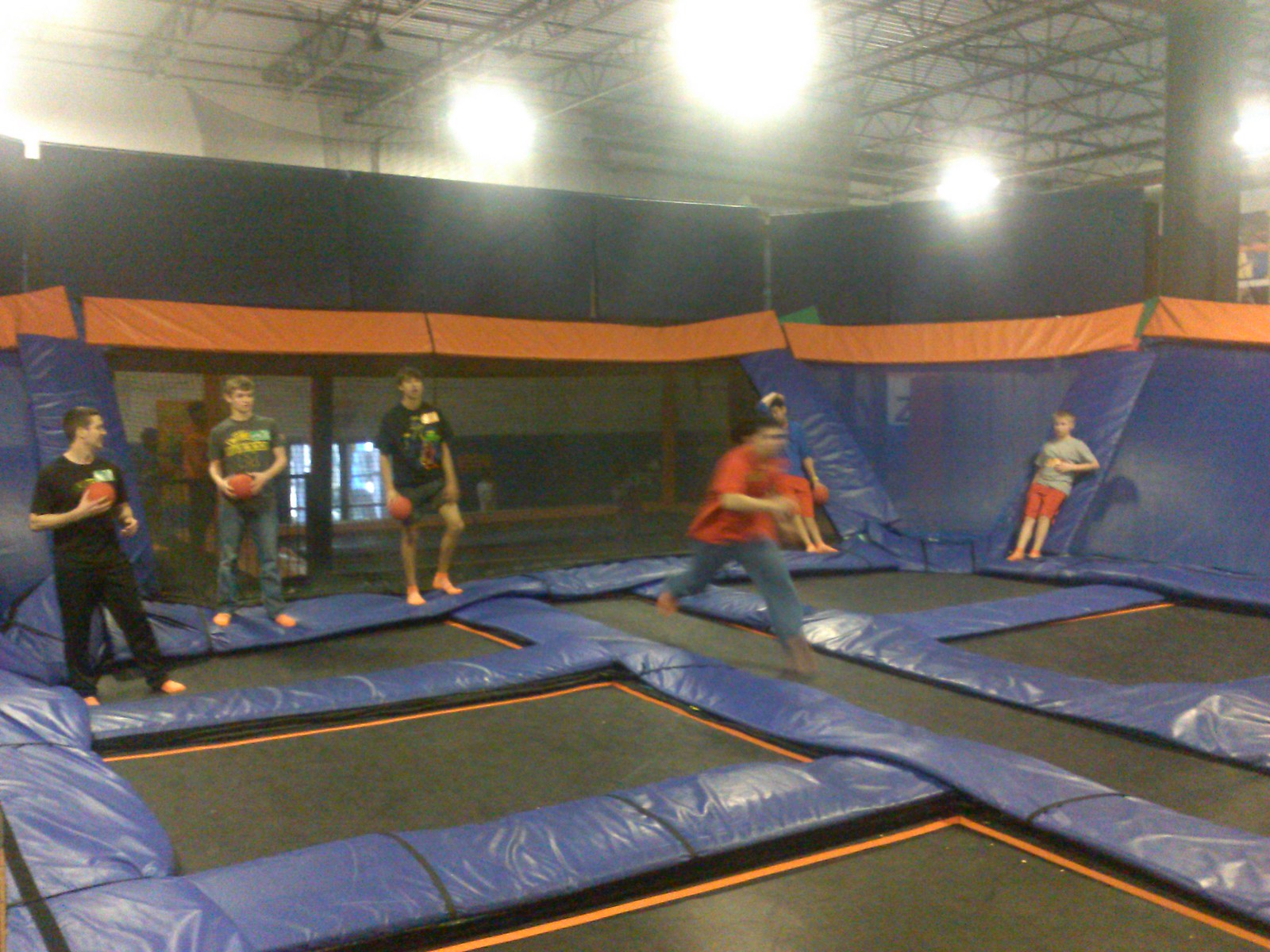The detailed indoor scene captures a lively moment in a large, hangar-like trampoline park characterized by a high ceiling adorned with powerful white lights and an extensive network of pipes. The room is accented by blue padded walls, with orange and blue tarp-like material covering sections of the walls and trampolines. The trampolines themselves are black and are divided by blue padded material, with an orange outline marking the top borders of this activity area. The floor is divided into rectangular sections, with a clear path running through the middle.

In this vividly lit setting are six teenage boys. Each is distinctively dressed: one in a black shirt with black pants, another in blue jeans and a gray shirt, one in shorts with a black shirt, another in blue jeans with a red shirt, one in red shorts with a blue shirt, and lastly, one in red shorts with a gray shirt. Five of these young men are stationary, holding small orange balls, positioned as though they are anticipating action. The sixth boy is caught in motion, running down the central aisle, his movement blurred, suggesting a game or chase involving the balls. The overall scene is energetic and engaging, capturing a dynamic moment within the expansive indoor venue.